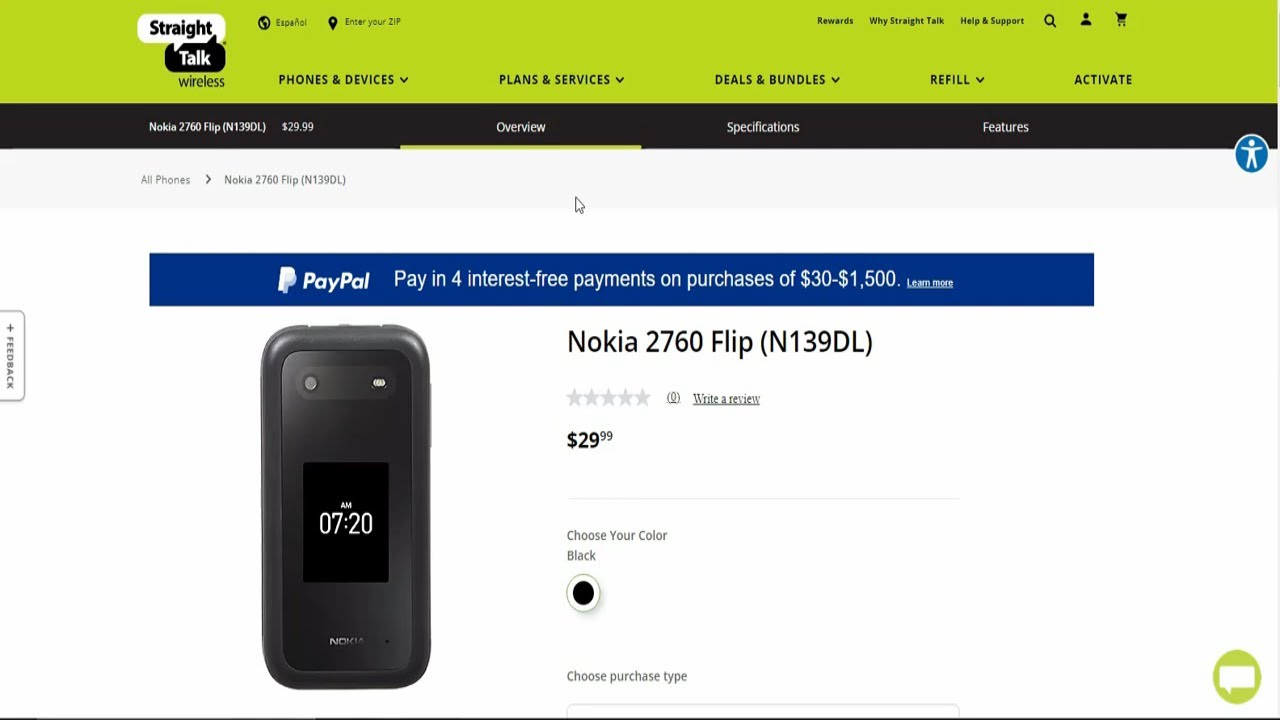This screenshot in landscape mode features a detailed layout of the Straight Talk Wireless website.

At the very top, a green navigation bar spans from the upper left to the upper right corner, prominently displaying the Straight Talk Wireless logo. The topmost row includes options for entering your zip code, accessing the rewards program, understanding why to choose Straight Talk, and getting help and support. Towards the right side of this row are icons for search, user account, and shopping cart functionalities.

Below this, a series of tabs are shown, indicating various categories such as "Phones & Devices," "Plans & Services," "Deals & Bundles," and "Refill & Activate." These are part of the navigation tools to explore the website offerings.

The next row features a darker background with a specific focus on the Nokia 2760 Flip phone, priced at $29.99. This section includes an "Overview" tab underlined in the signature green, highlighting it as the active selection. To the far right of this row, there are two additional tabs: "Specifications" and "Features." Additionally, there is an icon of a person inside a blue circle, presumably for contacting customer support.

Following this, a blue strip runs across the screen, promoting a special PayPal offer of interest-free payments on purchases ranging from $30 to $1,500.

On the left side of the screen, there is an image of the Nokia 2760 Flip phone displaying the time as 7:20 AM. Beneath this image, the text reiterates the price of $29.99 and includes an option to choose the color, which defaults to black.

The entire layout is designed to provide comprehensive information about the product and available services in a user-friendly manner, with crucial details and promotional offers clearly highlighted.